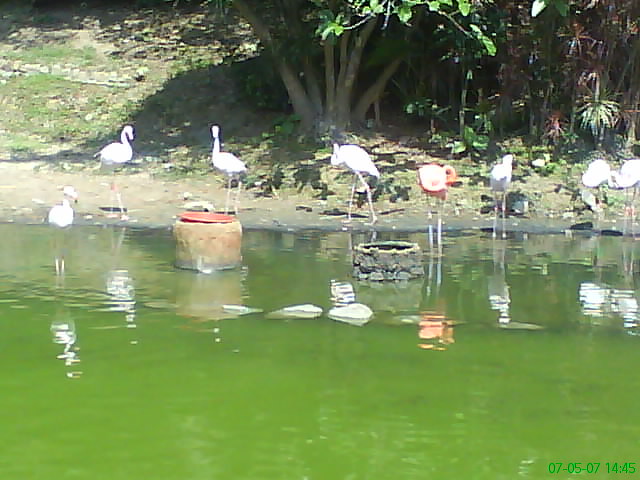This outdoor photograph, taken on a sunny day, captures a vibrant scene of numerous flamingos standing along the edge of a lime green, algae-tinged body of water, with their reflections mirrored in the surface. The water is framed by a light brown embankment and flanked by dense plants and trees with dark green, red, and green leaves. Among the flock of flamingos, one noticeable bird with long legs and white feathers stands on the left side towards the photograph’s edge. Prominently jettisoning out of the water is a large cylindrical structure, brown with a red top, and to its right, another structure resembling a well made of brown and gray bricks. Amidst these, a pink flamingo is seen elegantly curling its neck, forming a shape reminiscent of a candy cane. On the embankment itself, there are six white flamingos with their long necks either gracefully arched or extended. The ground is a mixture of tan soil and patches of green grass, with some smaller plants in the area providing a natural array of colors and textures. The overall tableau is marked by the serene and natural setting, accentuated by the vivid details of the birdlife and the surrounding environment.